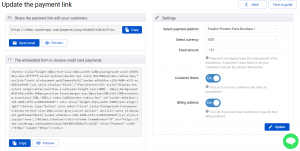This screenshot displays a small portion of a website dashboard. Prominently, at the top left corner, a section heading reads "Update the Payment Link," accompanied by two buttons outlined in blue on its right side. Below this, the interface is divided into two main columns. 

The left column contains two sections, each topped with a grey header bar. The upper section has two solid blue buttons and one button outlined in blue, while the lower section includes one solid blue button and one outlined in blue.

The right column features a single section with a grey header bar. This section includes two blue toggle switches positioned above a list of five items. Additionally, a circular green button, likely intended for initiating a chat, is located at the bottom right corner of the screenshot.